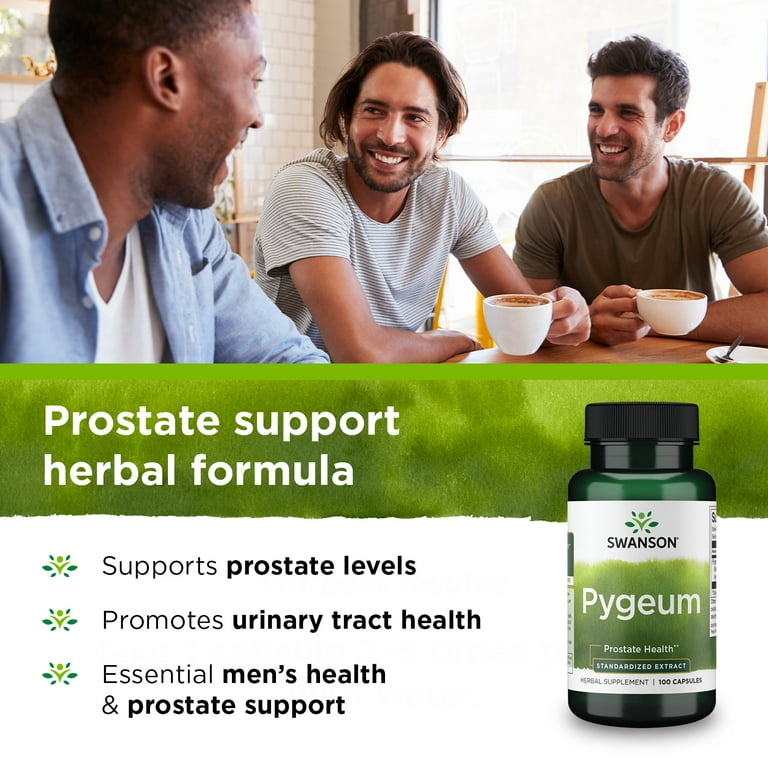The advertisement features three young men in a cozy coffee shop setting, sharing a light-hearted moment over white cups filled with brown liquid coffee. The men, showcasing diversity, consist of a black man in a blue denim shirt over a white V-neck tee, a Latino man with a green and white pinstripe shirt and long brown hair pulled back into a ponytail, and another white man, all engaged in a jovial conversation. The coffee shop’s ambiance is accented by a white brick wall on one side and large glass windows on the other, flooding the space with natural light.

Below this image, a prominent green horizontal stripe reads, "Prostate Support Herbal Formula," followed by three bullet points on a white background highlighting the benefits: Supports Prostate Levels, Promotes Urinary Tract Health, and Essential Men's Health and Prostate Support. To the right of these bullet points, a small dark green bottle with a black plastic lid and a white label that reads "Swanson Pygeum, Prostate Health" is displayed. The label also indicates that the bottle contains a standardized extract with 100 capsules, emphasizing it as an herbal supplement.